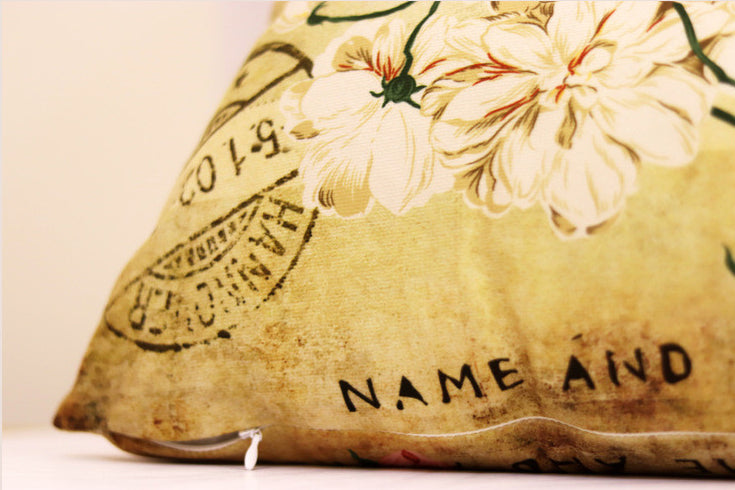This sepia-toned image captures a close-up view of a corner section of a pillow. The pillow, which appears to be light mustard yellow and somewhat dirty or faded, possibly due to wear or an artistic effect, prominently features floral designs with two cream-colored white flowers and green stems. Along the lower left edge of the pillow, a slightly open, small white zipper can be seen. Text is visible on the fabric, including the words "NAME" and "AND," alongside an upside-down circular stamp or logo that reads "Hanover 5102." The image focuses on the intricate details, providing a rustic, worn-out appearance and giving the impression that the pillow has been well-used or exposed to the elements.